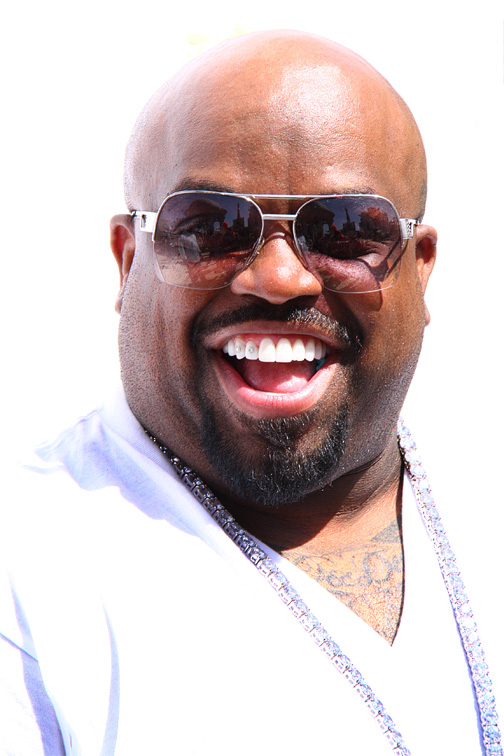In this image, we see Cee Lo Green, a black man with a bald head, who is smiling widely at the camera. He sports a short goatee and mustache, and is wearing a pair of sunglasses with stainless steel-colored frames. Some of his teeth, specifically on the left side, are adorned with jewels, visible due to his open-mouthed smile. Cee Lo Green is dressed in a light, V-neck top that appears white due to the intense lighting. This V-neck shirt reveals tattoos on his chest, including what seems to be the letter "D." Around his neck, he wears a prominent, purplish, or possibly silver diamond-encrusted necklace. The background of the photo is entirely white, enhancing the clarity and focus on him, and the image is oriented vertically, showing him from the chest up.